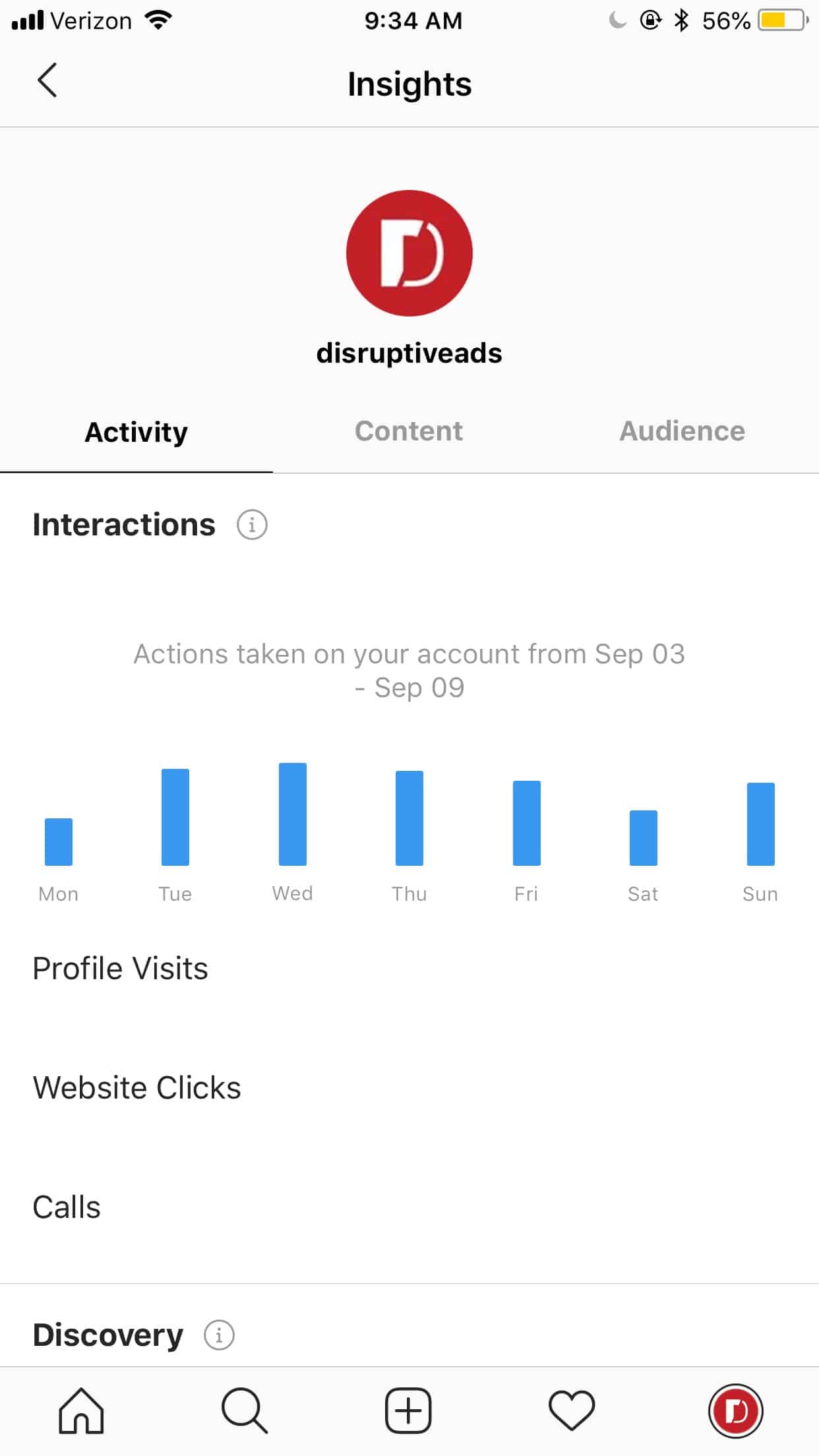This is an image of a smartphone screen. The battery life, marked in yellow, indicates 56% remaining and the device is connected to Verizon with a strong signal. The "Do Not Disturb" mode is activated, as shown by an illuminated moon icon. The current time displayed is 9:34 a.m.

At the top of the screen, the word "Insights" is prominently displayed. Below that, in the center of the phone, it reads "Disruptive Ads" within a large, round, red circle featuring a white 'D' in the middle. There are three selectable categories: "Activity," "Content," and "Audience." The "Activity" tab is currently selected, highlighted by a darker black background.

Underneath the "Activity" tab is a subsection titled "Interactions," accompanied by a small circle containing an 'i' icon. In lighter gray text, it states "Actions taken on your account from September 3rd to September 9th," and presents data in the form of blue bar graphs indicating levels of activity across days Monday through Sunday.

Further details include sections for "Profile Visits," "Website Clicks," and "Calls," with a heading labeled "Discovery" in dark black text. At the bottom of the screen, navigation icons are visible: a home icon, a search icon, a square with a plus sign, a heart, and the icon with a 'D' representing "Disruptive Ads."